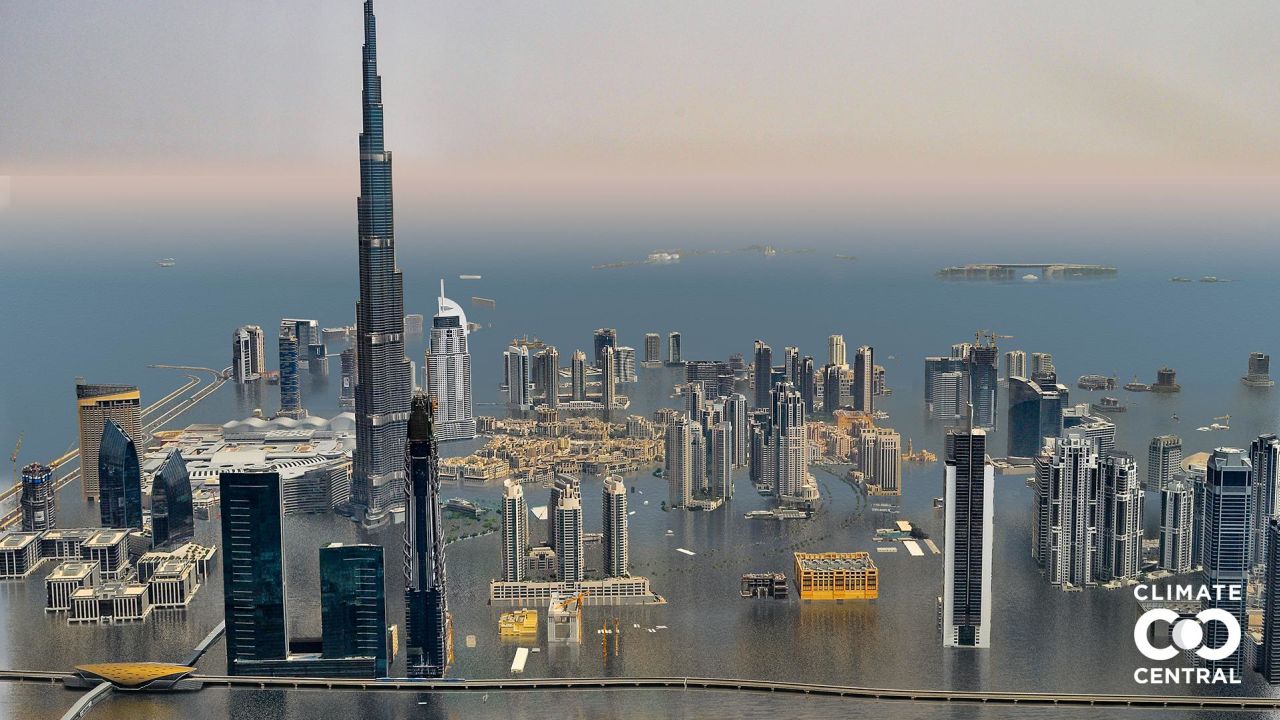The 3D rendering depicts a large, partially flooded cityscape with multiple skyscrapers. Dominating the scene is a very tall pointed tower, reminiscent of Dubai's Burj Khalifa, although specific identification remains uncertain. The city stretches across a rectangular frame, with the width being twice the height. Dark brown water inundates the lower sections of the city and extends into the horizon, where more buildings protrude from the floodwater. Notably, a road disappears into the engulfing waters on the left-hand side, and a possible rail system is visible along the bottom edge. The sky is a light gray, meeting an orange-tinted horizon line in the distance. In the bottom right corner, a logo displays “Climate Central” in white text, with a sideways figure of eight between the words.